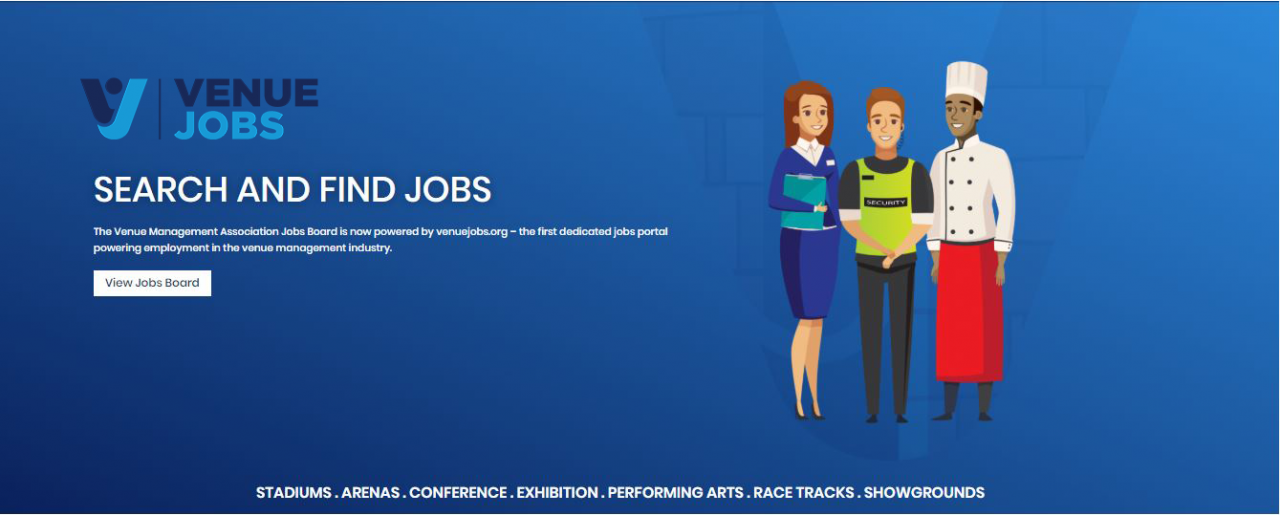A large blue rectangle featuring multiple elements, likely a graphic, banner, or magazine advertisement, dominates the image. In the top left corner, a logo is prominently displayed. This logo consists of a stylized 'V', with the left half in dark blue and the right half in light blue, centered by a dark blue dot. Just below the logo, a thin vertical blue line separates the text. To the right of this line, the word "Venue" appears in dark blue, and below it, "Jobs" is written in light blue.

Centered beneath the logo and text, large white letters boldly declare, "Search and Find Jobs." Directly below this, in smaller white lettering, an informative statement reads, "The Venue Management Association Jobs Board is now powered by ValueJobs.org, the first dedicated jobs portal powering employment in the venue management industry."

Further down, a prominent white rectangle with black text encourages viewers to "View Jobs Board."

On the far right side of the image, three cartoon characters are depicted in professional attire. The first character, a woman in a blue suit and white blouse, holds a blue clipboard in her right arm. The second character is a man in black pants and a short-sleeved black shirt with white trim, over which he wears a green bib-style vest adorned with an unreadable white bar label. The third character is dressed in a complete chef's uniform, which includes a chef's hat, a double-breasted white jacket, and a long red apron.

Running along the very bottom of the image, white text lists various venues, reading: "stadiums. arenas. conference. exhibition. performing arts. racetracks. showgrounds."